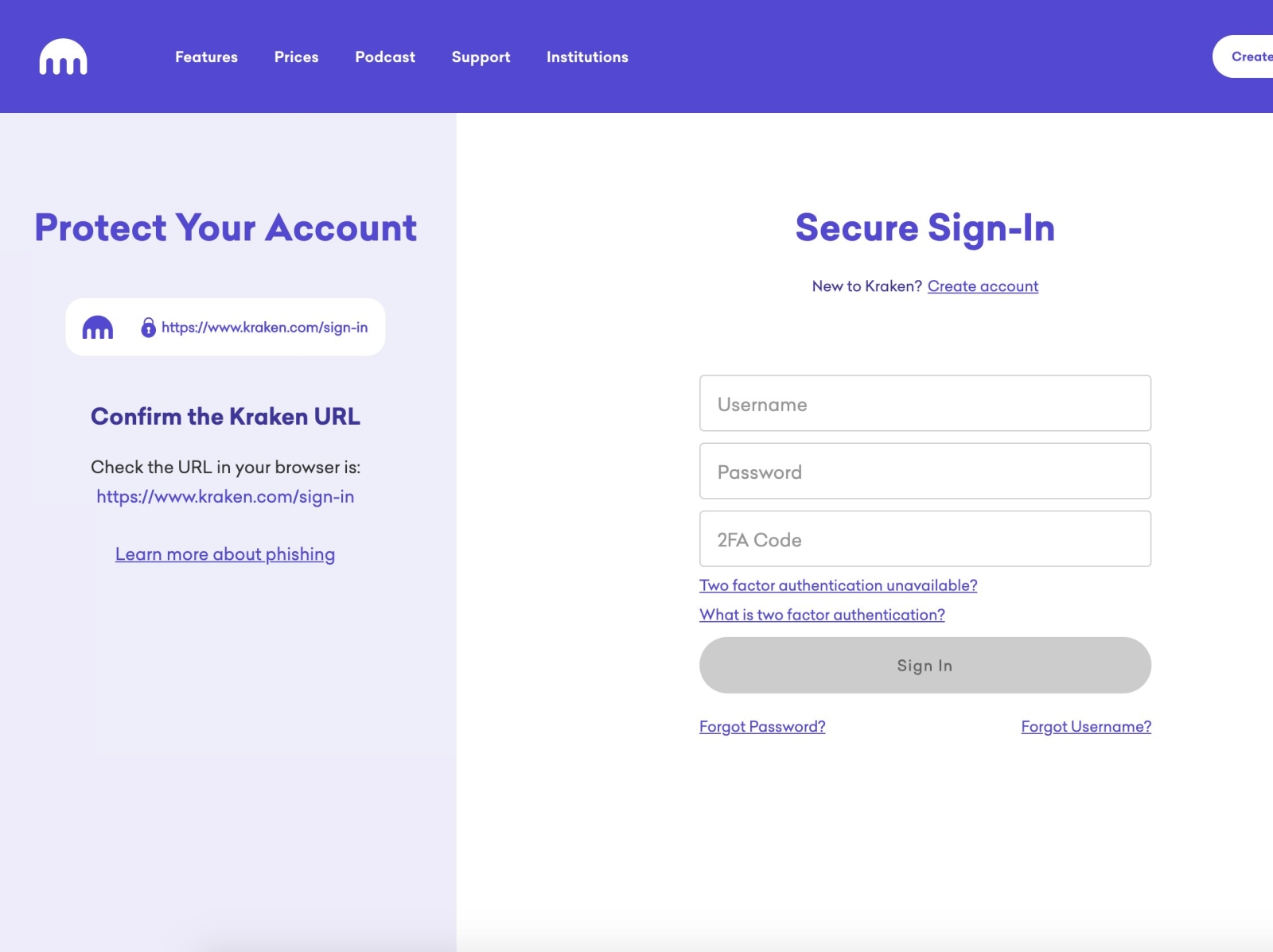This screenshot displays a website with a prominent purple banner at the top, featuring various navigational tabs that direct users to different sections. On the left side of the banner, there is a logo resembling a building with a circular top supported by columns, evoking the image of a traditional bank. The navigational tabs below the banner read "Features," "Prices," "Podcast," "Support," and "Institutions," indicating that this might be a website dedicated to podcasts, possibly with an educational focus.

On the top right corner of the banner, there is an option labeled "Create," suggesting that users can create their own podcasts on this platform. The left sidebar includes a notice prompting users to "Protect Your Account," accompanied by a link presumably directing to account security options. Just below, there's a message advising users to "Confirm the Kraken URL" by checking the URL in their browser, likely a security measure to ensure users are on the correct website.